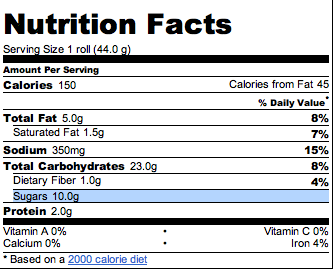A detailed image description of a Nutrition Facts label is prominently displayed. The header, "Nutrition Facts," is bold and black, making it easily noticeable. The label specifies that the serving size is one roll, indicating the nutritional information pertains to a single roll. 

The label reveals that one roll contains 150 calories, with 45 calories derived from fat. The total fat content is 5 grams, which constitutes 8% of the daily recommended intake. Out of this, saturated fat makes up 7%. Sodium content is listed as 350 milligrams, amounting to 15% of the daily value. Total carbohydrates are at 8%, with dietary fiber making up 4% and sugars at 10 grams. The protein content is 2 grams. 

The vitamin and mineral content is minimal with Vitamin A, Vitamin C, and calcium all at 0%, whereas iron is at 4%, all based on a 2,000 calorie diet. The image solely features the Nutrition Facts label without any accompanying picture of the roll itself.